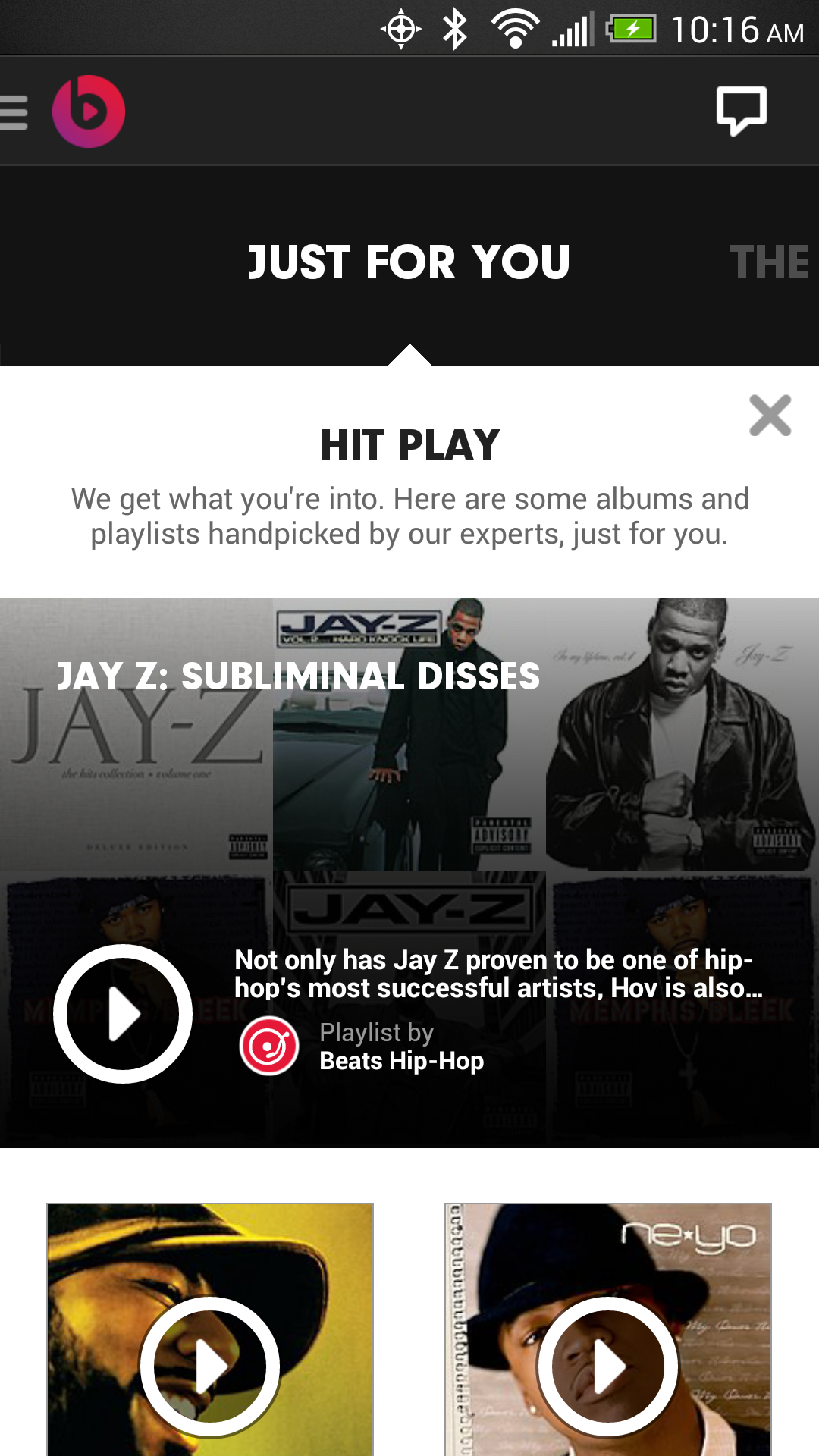This image showcases an old interface of Beats Music's streaming service, a competitor to Apple Music before its acquisition by Apple. The screenshot, evidently from a smartphone, features the Beats Music logo prominently. 

The interface is organized with a menu icon on the left, providing access to various sections of the service. A standout feature is the "Just for You" section, which suggests hand-picked playlists and albums tailored to the user’s tastes, leveraging data algorithms for personalized recommendations. 

On display are album covers from renowned artists such as Jay-Z, Common, and Ne-Yo, each with visible play buttons, encouraging immediate engagement. Notably, there’s a marquee note about Jay-Z, highlighting his significance in hip-hop, alongside curated playlists labeled “Hip-Hop,” confirming the app’s commitment to genre-specific content.

The caption encapsulates a historical glimpse into the user experience of Beats Music, reflecting its design and features aimed at music discovery and personalization before its evolution into what is now Apple Music.